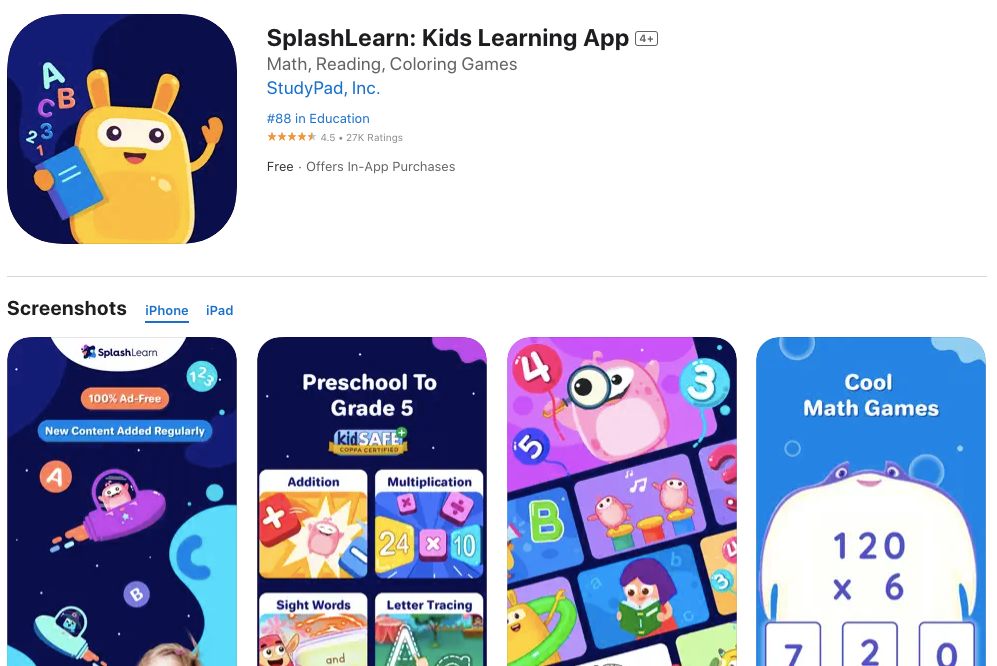The image shows a website featuring educational games for children. At the top of the page, a cheerful yellow creature with antenna-like ears waves while holding a book, with "ABC" and "123" displayed beside him. The banner reads "SplashLearn: Kids Learning App," followed by the text "Math, Reading, Coloring Games." The app is created by StudyPad, Inc. and is ranked #88 in the Education category. It boasts a star rating of 4.5 from 27,000 ratings. The app is free to download, with optional in-app purchases available.

The lower section of the image includes four screenshots showcasing different aspects of the app for iPhone and iPad. The first screenshot highlights that the app is 100% ad-free and features new content added regularly. It states that it caters to children from preschool to grade five within a kid-safe environment. Various educational activities are displayed, including a box for addition, a box for multiplication, a sight words box, and a letter tracing box. The second screenshot features animated characters and letters, while the third screenshot promotes "Cool Math Games."